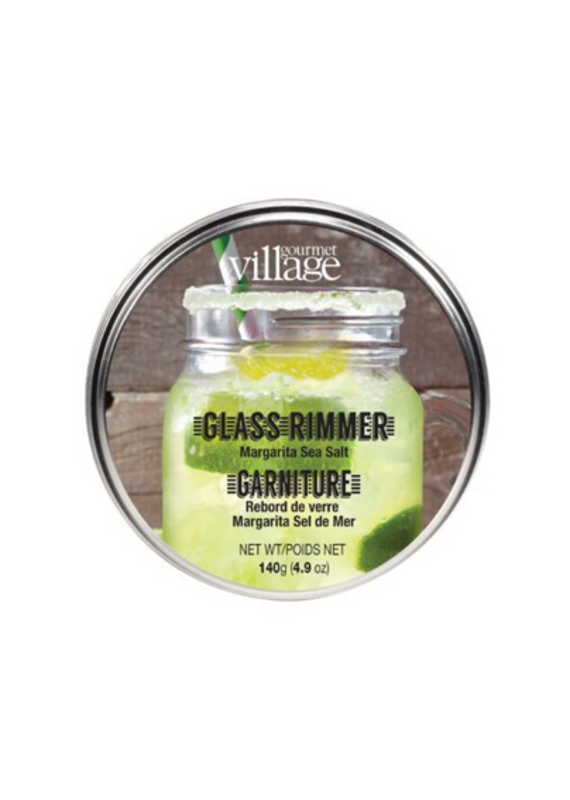The image features the lid of a round metallic tin of Gourmet Village's Glass Rimmer Margarita Sea Salt. The lid displays a vivid picture of a jar filled with a green margarita, garnished with a few lime wedges and a green and white straw. The margarita glass has a salted rim, accentuating its refreshing appeal. Text on the lid includes "Gourmet Village" at the top in white letters, and "Glass Rimmer Margarita Sea Salt Garniture," along with additional information in a different language. The net weight, 140 grams or 4.9 ounces, is also specified. The tin appears to be set against a wooden backdrop, enhancing its rustic charm.